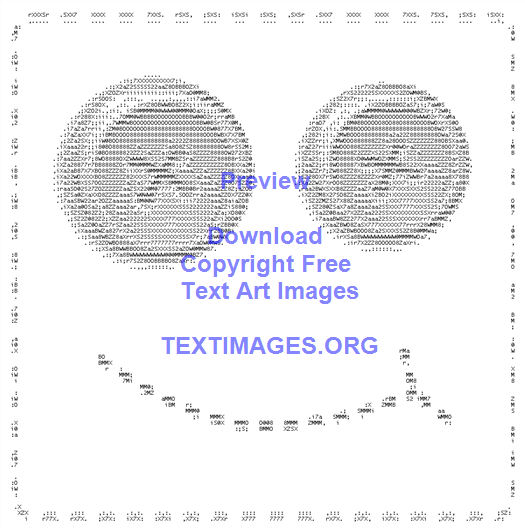The image is a cropped graphic from textimages.org, featuring a square composed primarily of ASCII art. At the center of the square, a smiley face is depicted with large, round eyes that resemble sewed buttons, each eye marked with an X to indicate the pupils. Below the eyes, a smile stretches across the face, consisting of a simple line with an additional line at the right end, forming an unmistakable happy expression. Overlaying the graphic is a blue watermark with the text: "Preview Download Copyright-Free Text Art Images" from textimages.org. The overall design suggests an advertisement for a website offering downloadable ASCII art and other text-based images.